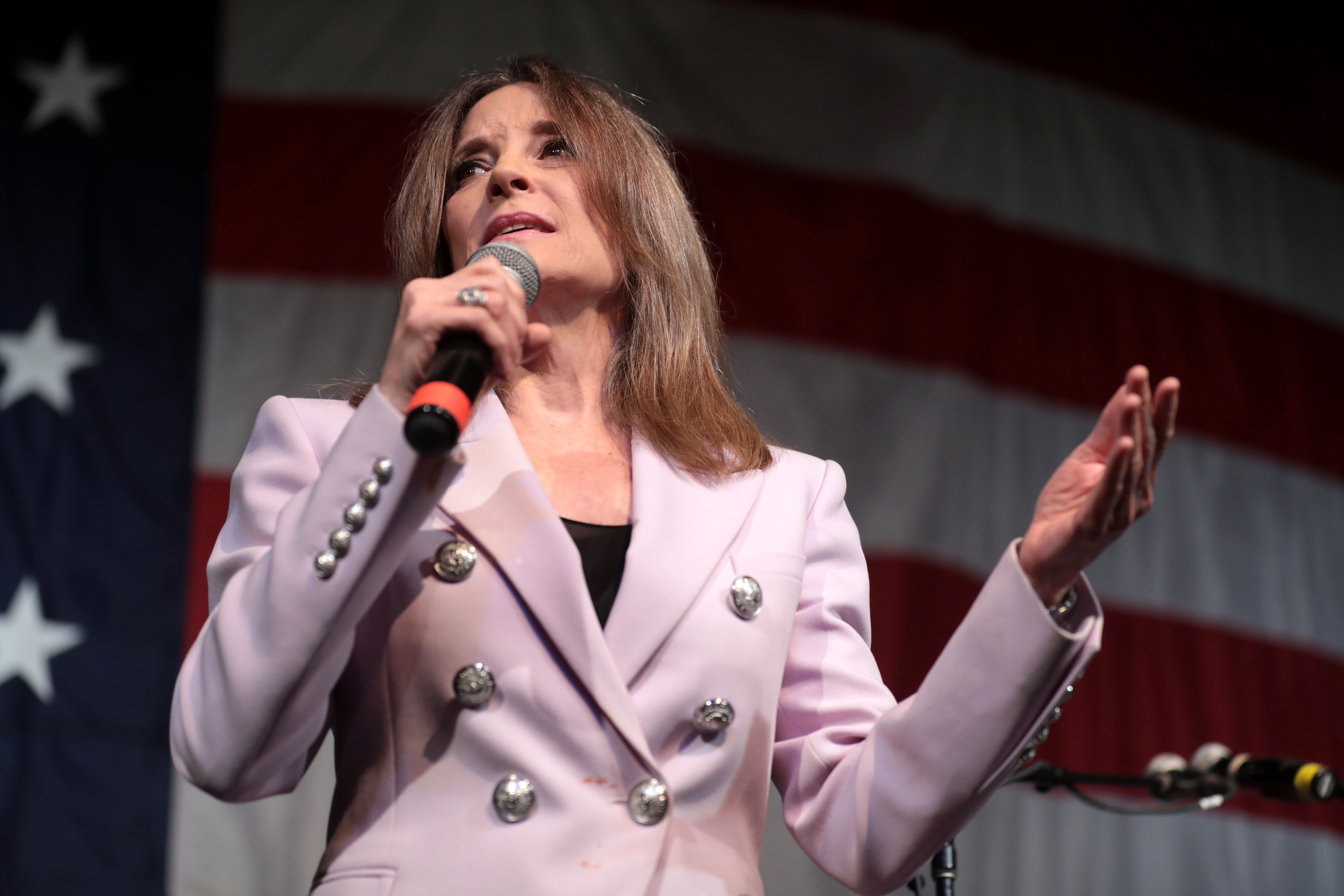Photograph of a woman, likely a politician in her 40s or 50s, on a stage giving a speech. She is at the center of the frame, holding a black microphone with a silver top in her left hand, appearing mid-speech or perhaps pausing. The backdrop features a large American flag. The woman has shoulder-length brown hair and is dressed in a lilac blazer with multiple silver buttons—six on the front, with only one button fastened, and five buttons on each sleeve cuff. She wears a black top underneath the blazer. A second black microphone, identical to the one she holds but marked with yellow, is positioned on a stand to her right. The image appears professionally taken, given its close-up nature, good lighting, and sharp focus, suggesting it captures a moment from a political event, possibly a campaign fundraiser or similar gathering. Colors in the image include red, white, blue, black, white, off-white, beige, orange, pink, taupe, and yellow.